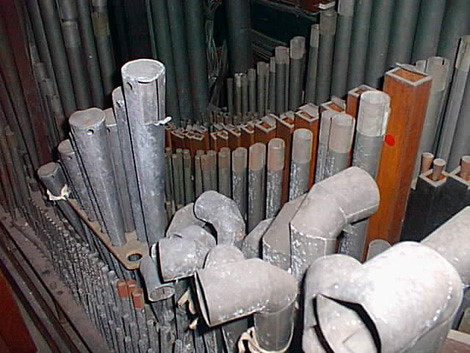This overhead, slightly front-angle photograph vividly captures a dense array of organ pipes in a strikingly industrial, dusty setting, offering a glimpse into the intricate, seldom-seen interior of a pipe organ. The pipes, varying in shape and size, are meticulously arranged in semi-circular rows that span from short to tall as they fan out to the right and then tall to short towards the left, creating an almost rhythmic visual pattern. The pipes exhibit a dusty, tarnished silver appearance, adding to the sense of aged neglect. Thin, silver pipes dominate the foreground, with three distinct ones sporting orange tape around their tips, hinting at possible repairs or replacements. In the middle of the composition, approximately six slender, silver pipes rise slightly upward, while the bottom right corner is densely packed with about twenty aluminum pipes, each curving at the top to form noticeable elbows. Behind these, more silver pipes descend diagonally, some wrapped in brown tape, leading the eye further into the depth of the image. Square, brown-tapered pipes further enrich the scene, contributing to the array's complexity. Towards the back, bundles of pipes, some ascending off the screen, reinforce the organ's grand scale. This detailed assembly suggests a purpose beyond mere industrial function, possibly linked to the restoration or maintenance of the organ, evoking a compelling blend of artistry and mechanics.